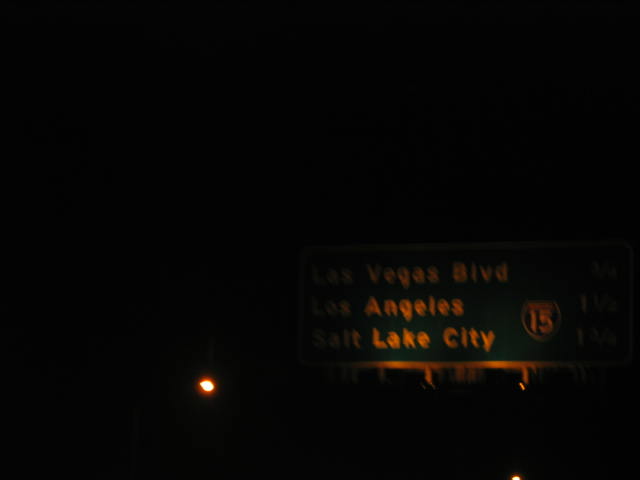This is a nighttime photo taken, presumably from a car, of a freeway sign on a dark road. The image is predominantly pitch black, save for a dimly lit green highway sign in the right middle section of the picture. The sign, partially illuminated by what appear to be headlights, displays "Las Vegas Boulevard," "Los Angeles," and "Salt Lake City" in white letters, along with a highway logo marked "15." The letters "Las Vegas Boulevard" are abbreviated as "B-L-V-D" and the words "Los Angeles" and "Lake City" are the most visible under the limited light. The sign appears to be hanging overhead, viewed from a low perspective, and blends into the dark background. Additionally, there is an orange-yellow light in the distant background to the left of the sign, whose source is ambiguous. The image creates a stark contrast between the illuminated sign and the surrounding darkness.